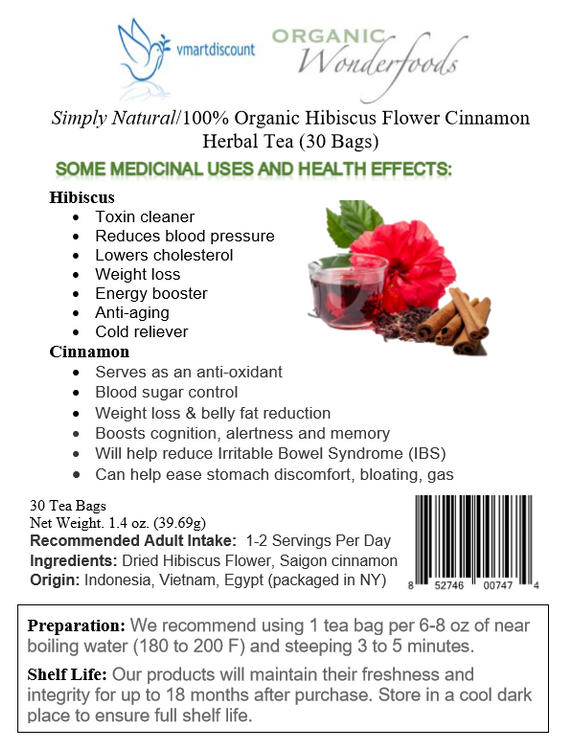The image depicts a detailed label or advertisement for "Simply Natural 100% Organic Hibiscus Flower Cinnamon Herbal Tea," featuring logos for "V Mark Discount" and "Organic Wonder Foods" at the top. Central to the design is a small picture of a bird with an olive leaf. Below the tea name, in bold green font, are medical uses and health effects of the ingredients. 

For hibiscus, the benefits include: toxin clearing, reducing blood pressure, lowering cholesterol, supporting weight loss, boosting energy, anti-aging properties, and cold relief. For cinnamon, the benefits listed are: antioxidant properties, blood sugar control, weight loss and belly fat reduction, cognitive alertness and memory enhancement, and easing stomach discomfort from bloating and gas.

On the right side, the label includes an image of a clear glass cup filled with a dark red liquid, presumably the tea, set against a backdrop of a vibrant red hibiscus flower and complemented by ground and stick cinnamon. The label confirms the product contains 30 tea bags and lists preparation instructions, shelf life, ingredients, product weight, origin, and a barcode on the right side. The text is predominantly in black against a white background, emphasizing clarity and readability.